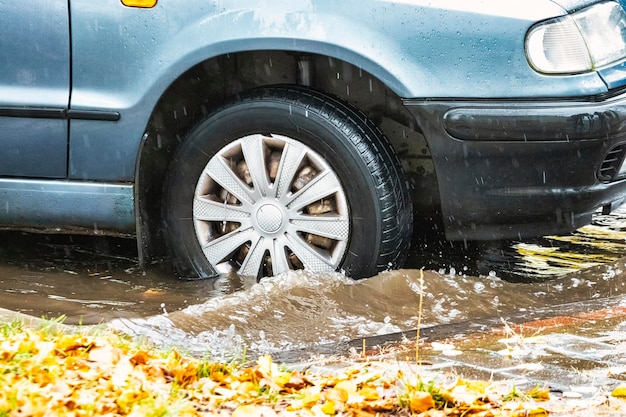In this detailed image, we see the close-up of a teal blue car, specifically the front passenger side, including the headlight, part of the hood, bumper, and the right front wheel. The vehicle's distinctive rims feature an unusual check pattern which might suggest they are custom made. The scene captures the car navigating through several inches of standing, brown and murky water, possibly indicating flooding or heavy rain. This moment, taken from a wide landscape perspective, shows the water with small waves, implying an ongoing downpour. Additionally, there are autumn leaves in shades of red, yellow, and orange scattered at the bottom of the image, hinting at the fall season. Behind the car, a bit of grass is visible by the sidewalk, adding to the context of the surroundings.